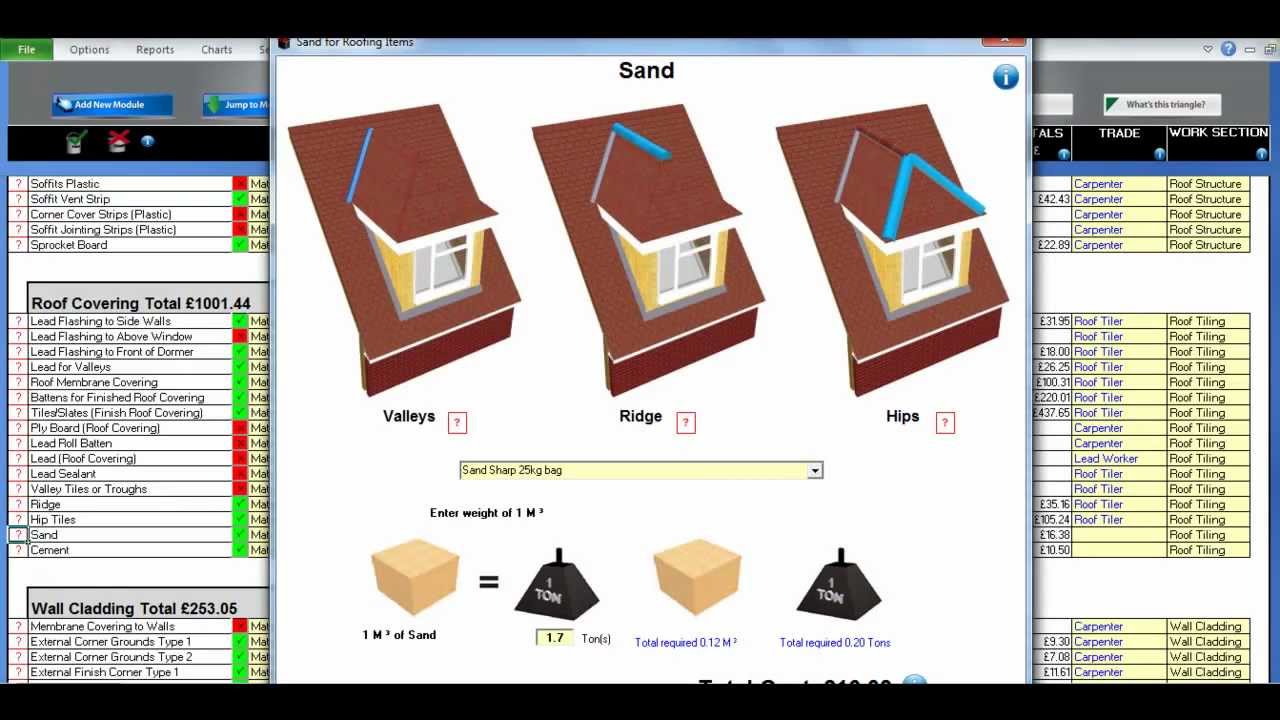The image is a photograph of a computer monitor displaying a detailed Excel spreadsheet related to roofing planning for a house. In the center of the screen, there's a distinct pop-up that features three drawings of a section of a roof, each with specific areas highlighted in light blue. The first drawing highlights the area around a window and labels sections as "valley," "ridge," and "hip." Below these drawings, there is a label "sand for roofing items," and details such as "1 meter cubed of sand equals 1.7 ton total required" and further conversion notes.

Additionally, the pop-up contains visual representations like a cardboard box labeled "sand sharp 25 kg bag," and a pyramid-shaped weight indicating "1 ton." The spreadsheet background shows comprehensive tabulated data. Prominent titles include "roof covering total," which is listed as £1001.44, and "wall cladding total," marked as £253.05. There are various sections highlighted in blue, green, and red, indicative of different statuses or categories, with additional details and smaller text that provide further breakdowns of the roofing materials needed.